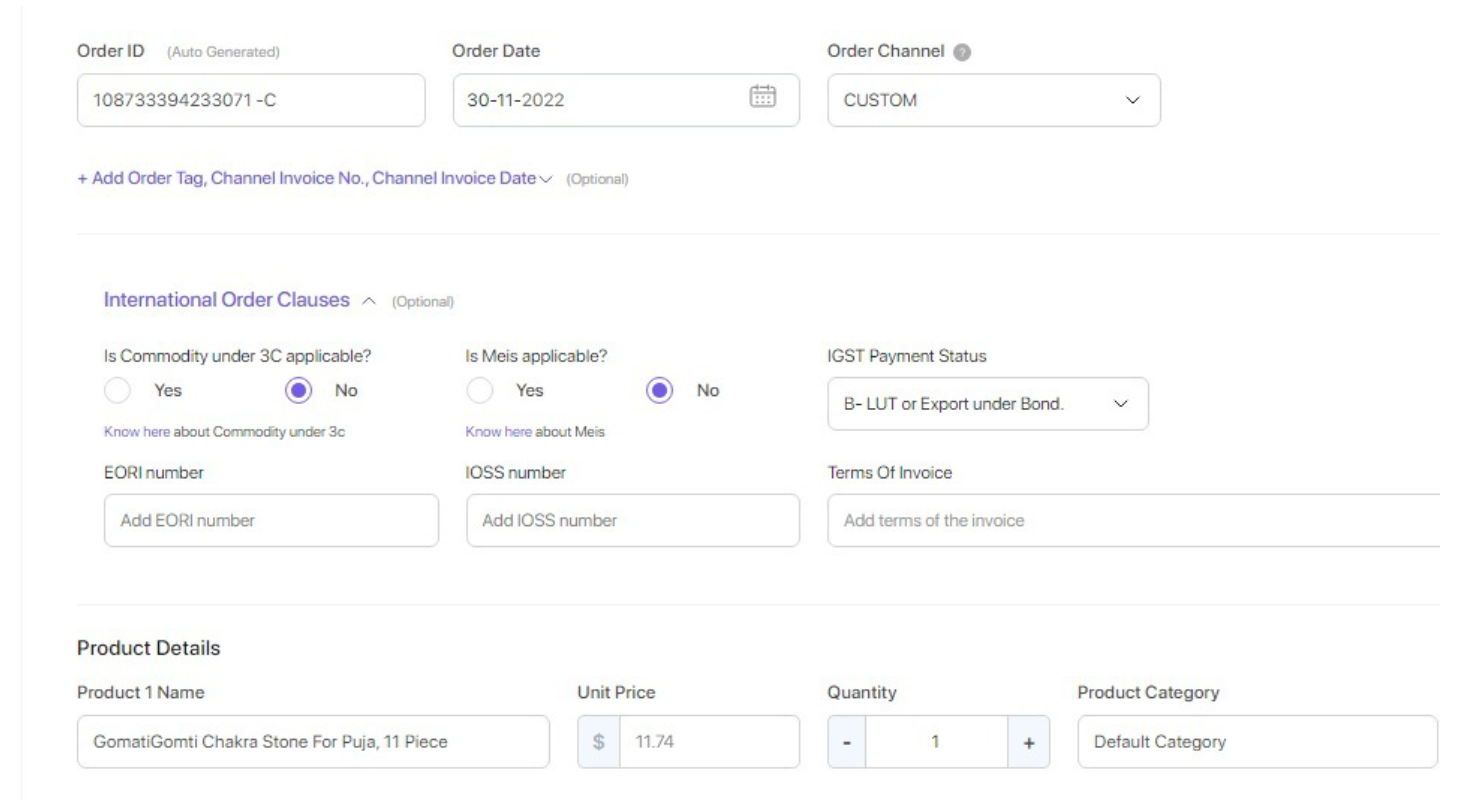This screenshot appears to be from a detailed commercial shipping form. The form is designed for business or commercial customers and appears more comprehensive than standard, non-commercial forms. Although the form lacks a title, suggesting it might be a portion of a larger document, it starts by requesting the order ID, which in this instance is auto-generated. The form also asks for the order date, specified as sometime in 2022, and the order channel, which is set to "custom." Additionally, users can add an order tag, channel invoice number, and channel invoice date.

Following this, the form includes an optional section for international order clauses. Despite being optional, this section has been filled out, with queries such as "Is commodity under 3C applicable?" and "Is MEIS applicable?" answered with "no." Notably, there are clickable buttons next to each question for users to select "no" for commodity under 3C and MEIS applicability. The form's language appears slightly awkward, indicating it may have been translated.

To the right of the international order clauses section, the IGST payment status is displayed as "B-LUT" or export under bond, which has been selected. The form also allows for the inclusion of an EORI number, an IOSS number, and the terms of the invoice.

The final visible section on the screenshot contains product details. It lists "Product One" as "Gomati Gomti Chakra Stone for Puja, 11 piece," priced at $11.74 per unit, with a quantity of one. The product category is set to the default category. The product name, "Gomati Gomti Chakra," and the word "puja" (meaning ritual worship in Hindi), suggest that this form could be from an Indian or South Asian website or business platform.